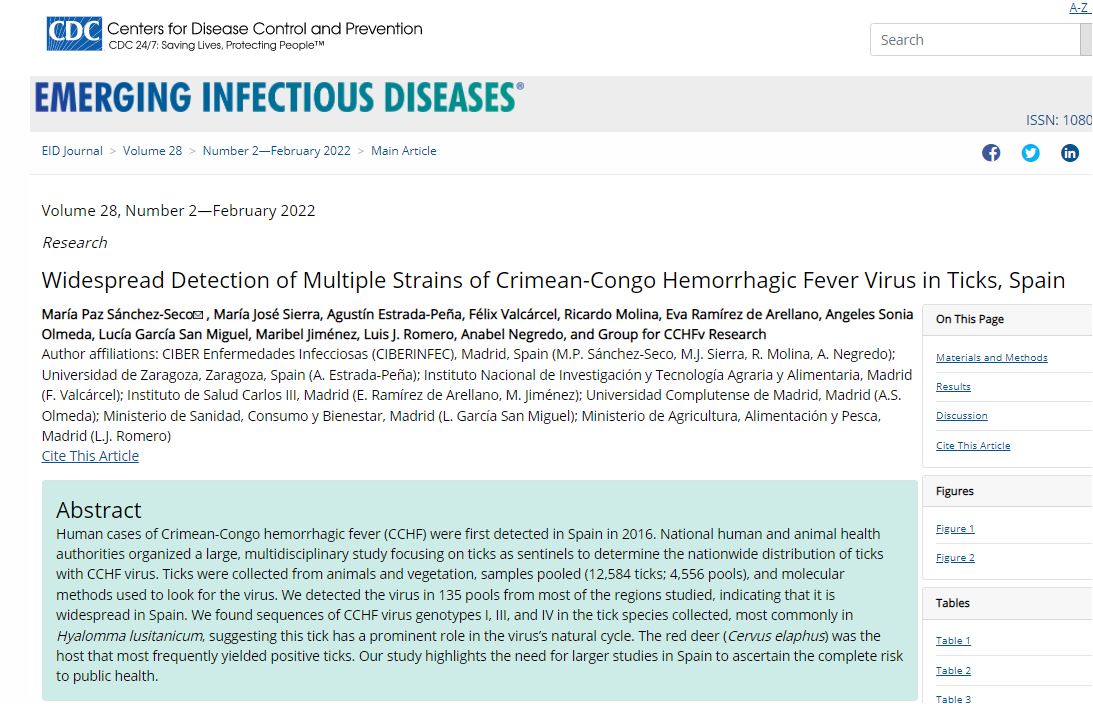This rectangular image depicts a web page from the official website of the Centers for Disease Control and Prevention (CDC). The long side of the rectangle runs horizontally from left to right. At the top of the page is a white border with the CDC logo prominently displayed on the upper left-hand side. Just below this, the slogan "CDC 24/7: Saving Lives, Protecting People" is included.

A light gray border follows right underneath the white section, segmented by text in bluish-green font reading, "Emerging Infectious Diseases." Below this title, the text continues with "EID Journal Volume 28, Number 2 - February 2022, Main Article."

Further down, in another clearly defined section, the text reads "Volume 28, Number 2 - February 2022, Research," followed by an article title: "Widespread Detection of Multiple Strains of Crimean-Congo Hemorrhagic Fever Virus in Ticks in Spain." Below this section, the document likely elaborates on the findings described.

At the bottom of the image, there is an abstract highlighted in turquoise, offering a summarized overview of the research issue. This detailed layout effectively structures the webpage with sections organized by their respective headings and content focus.